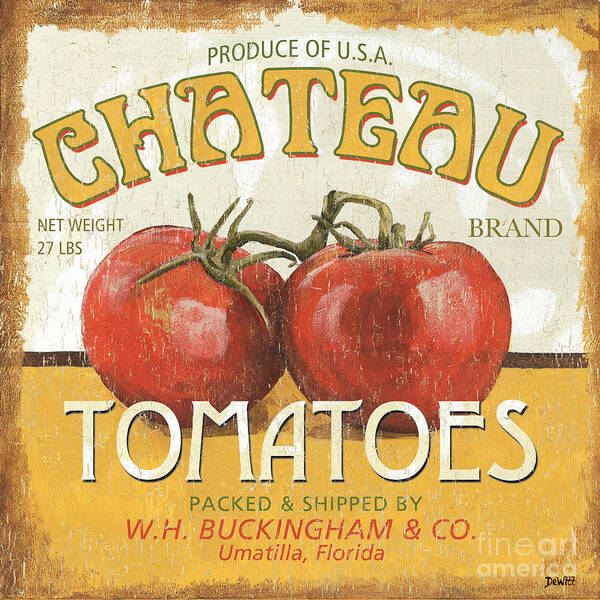The weathered image portrays an old produce label with a brown periphery. At the top, it features "Produce of USA" in green lettering. Below that, "Chateau" is prominently displayed in large, yellow letters outlined in green. The center of the label showcases two vivid red tomatoes still connected by their green vine, resting on a gold tabletop. To the left of the tomatoes, it specifies "Net Weight 27 pounds," and to the right, it notes "Brand." Beneath the tomatoes, "Tomatoes" is written in capitalized white letters, followed by "Packed and shipped by W.H. Buckingham and Co., Umatilla, Florida." The image is clear and well-lit, with a watermark reading "Fine Art America" located in the bottom right corner.